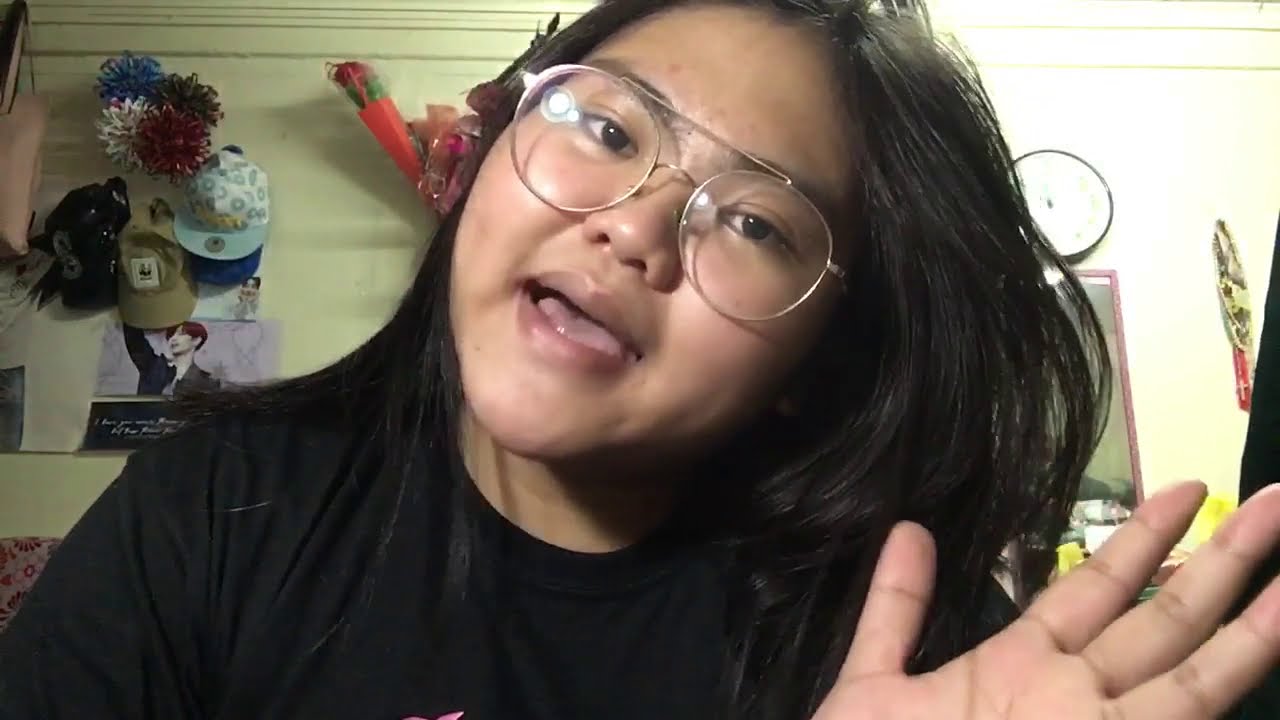The image captures a young girl, possibly of Indian or Asian descent, seated in front of the camera with an engaging gesture of waving her left hand. She appears to be around 14 or 15 years old, sporting long black hair that cascades down past her shoulders, and is wearing large, black metal-rimmed glasses. Her head is tilted to her right, and her mouth is slightly open as if she's speaking to the camera. She is clad in a black short-sleeved t-shirt featuring a design that is mostly cropped out, but you can see a hint of pink from it.

She is positioned against a background of a beige or greenish-yellow wall adorned with an array of decorative items. To her left, the wall is decorated with a variety of hats: a black hat, a green hat, a dark blue hat, a white hat with a light blue brim, and a possibly dark or light brown hat. Above these hats, there are colorful pom-poms or bows in shades of red, white, blue, and gold. Among the decorations is a K-pop poster featuring a young man with red hair. 

On her right side, there's a round clock with a white face and a black outline, positioned above a vertical mirror framed in pink or red. Adjacent to the mirror, there's a red flower in a red container adding a pop of color to the scene. The overall setting suggests it's probably her bedroom, with personal and decorative touches adding to its lively atmosphere.